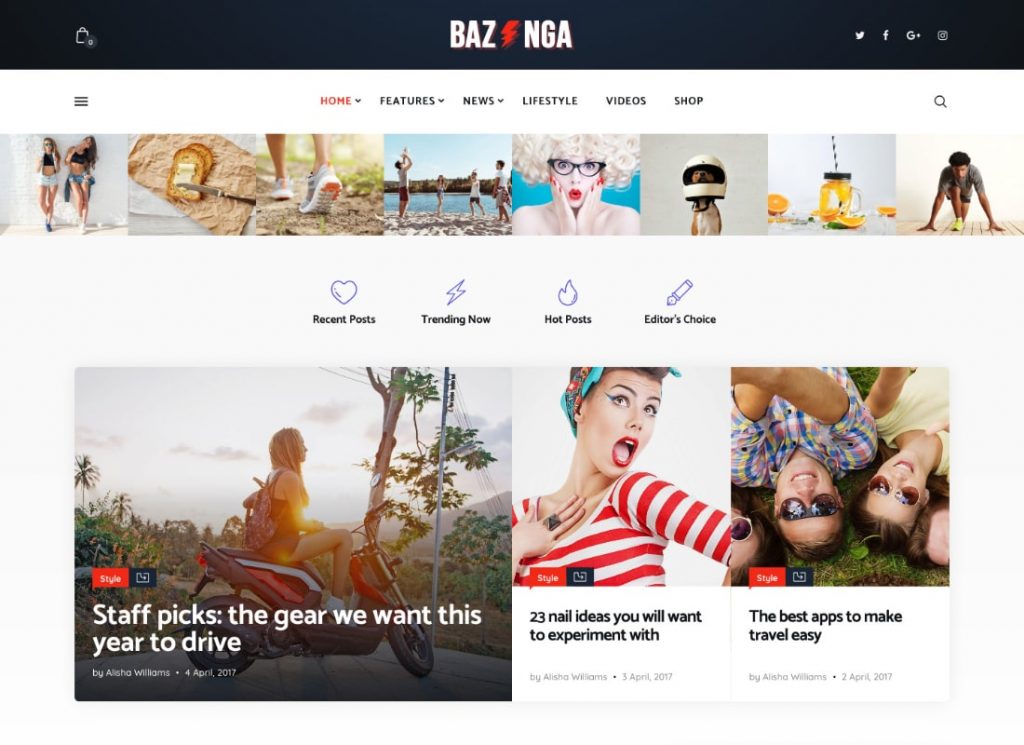**Detailed Caption for Bazinga Screenshot:**

The screenshot captures the Bazinga webpage, characterized by a prominent black bar spanning across the width of the screen. In the center of this bar, the word "BAZINGA" is displayed in bold, capitalized white text, with a striking red lightning bolt interjected between "BAZ" and "NGA." 

Positioned in the top left corner of this bar is an outlined white lock icon with a number "0" noted at its bottom right. On the opposite end, to the right of "BAZINGA", there are icons for social media platforms in white – Twitter, Facebook, Google Plus, and Instagram. 

The background is light gray, complementing the navigation bar at the top of the page. This navigation bar is designed with a black "hamburger" menu icon on the left, followed by menu options in different styles: "HOME" in bold red capital letters with a drop-down arrow, while "FEATURES, NEWS, LIFESTYLE, VIDEOS," and "SHOP" are all in black capitals, each with their respective drop-down arrows. Concluding the menu list on the right side is a white magnifying glass icon, implying a search function.

Below the navigation bar is a series of images, formatted into a visual strip. The first picture features two girls leaning against a white wall. Both have long, flowing hair; the girl on the left with lighter hair wears glasses and black tank top, adorned with a button-up shirt over it, white jean shorts, and a pair of black or blue sneakers. She is striking a casual pose with her right leg bent, foot against the wall, and standing on her left foot. The girl on the right, with darker hair, stands with her head tilted, her right hand up near her face, wearing black jean shorts and a dark-blue shirt draped over her shoulder. She is also leaning against the wall with her right leg bent behind her.

The subsequent images portray:
1. Two pieces of toast on a brown napkin placed over a piece of white paper atop a white surface, with a knife spreading butter on one toast.
2. A person walking on a dirt trail in the woods, shown only from the feet up to the mid-calf, wearing gray sneakers with a striking white, gray, and orange sole.
3. Four people engaging in a beach volleyball game, with an expanse of water and sandy shore visible behind them.
4. A zoomed-in shot of a pale woman with bleached blonde, afro-style hair, adorned with black glasses in a cat-eye frame, red lipstick, and a dramatic, surprised expression with her hands pressed to her cheeks, set against a teal background.
5. A dog wearing a small white helmet with a black interior, showcasing his tan face and dark features.
6. A photo of a glass jar with a handle and black lid, surrounded by orange wedges and half an orange, with a black and white striped straw.
7. A dark-skinned man poised to take off running, dressed in a gray shirt, yellow sneakers, and unspecified shorts, on a wooden floor against a white wall.

At the bottom of this section is a wide white area segmented into four categories: "Recent Posts" with a blue heart outline, "Trending Now" with a blue lightning bolt outline, "Hot Posts" with a blue flame outline, and "Editor's Choice" with a blue pen outline.

Centered below is a large picture occupying half the space, depicting a woman with a backpack seated on a motorcycle. The bike features a black seat with white and red striping, set against a scenic background of distant mountains, a utility pole, and surrounding vegetation. The image includes a red box labeled "STYLE" in white text, and a black box with a white outline next to it, followed by the bold white text "STAFF PICKS: THE GEAR WE WANT THIS YEAR TO DRIVE" and the byline "By Alicia Williams, 4 April, 2017."

To the right are two more images. The first shows a woman with a white and red striped shirt, hands over her chest, mouth open in an exclamation, and sporting a blue floral headband and red lipstick. Accompanying text includes a red box labeled "STYLE" and the title "23 Nail Ideas You Will Want to Experiment With" by Alicia Williams, dated 3 April, 2017. The second image captures four people lying on the ground taking a selfie, one of whom is a man in a colorful checkered shirt, set under the same format with the title "The Best Apps to Make Travel Easy" by Alicia Williams, dated 2 April, 2017.